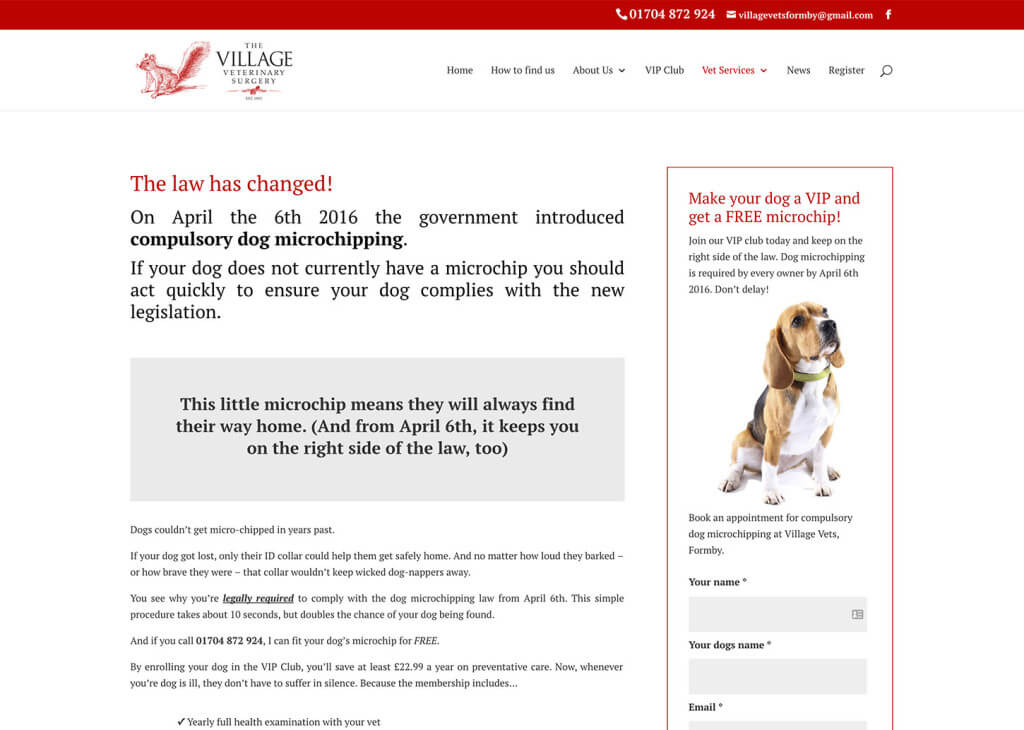**Detailed Caption for the Screen Capture:**

The image is a screen capture from a veterinary website, prominently featuring a red banner at the top with white text. The banner includes a phone icon followed by the phone number "017-04-872-924", an email icon (represented by a white envelope), and a Facebook icon. Below this banner, there is an illustration of a bushy-tailed squirrel in red, accompanied by the text "The Village Veterinary Surgery" in black.

The navigation bar beneath the illustration includes several clickable submenus in black font: "Home", "How to Find Us", and "About Us". The currently hovered submenu has a white mouse cursor over it, making the text indistinguishable. Another submenu, "Vet Services" in red, has a down arrow next to it, followed by other submenus in black such as "News" (indicated by the word “black” mistakenly interpreted as a section title) and "Register". The navigation bar also features a black magnifying glass icon.

The main content area starts with a notice in red reading, "The law has changed". This is followed by black text detailing that as of April 6, 2016, the government requires compulsory microchipping for dogs. The text emphasizes the legal requirements and benefits of dog microchipping, including enhancing the chances of recovering lost pets and deterring dog theft.

A grey box with black text inside says: "This little microchip means they will always find their way home. And from April 6th, it keeps you on the right side of the law too." The box continues with the historically challenging aspects of lost dogs, stressing the importance of the new legislation by saying: "You see why you're legally required to comply with the dog microchipping law from April 6th." It further explains that the microchipping procedure is quick, taking about 10 seconds, and it doubles the likelihood of a lost dog being found. There's an offer to fit a microchip for free if you call the provided number.

The page highlights a promotion for the "VIP Club", which promises savings on preventative care and yearly check-ups with a vet, noting benefits and an offer for membership.

To the side, there is another red banner urging users to "Make your dog a VIP and get a free microchip". The banner includes additional details about the VIP club and legal compliance by April 6, 2016.

An image of a tan, white, and black dog wearing a gold-olive collar is featured below, captioned with "Book an appointment for compulsory dog microchipping at Village Vets, Thornby". Below this, a form for appointments is visible, with labeled boxes for user information: "Your name," "your dog's name," and "email," each marked with an asterisk denoting required fields.

Overall, the screen capture presents important information, legal requirements, promotional offers, and practical steps for ensuring pet safety and compliance with new laws.